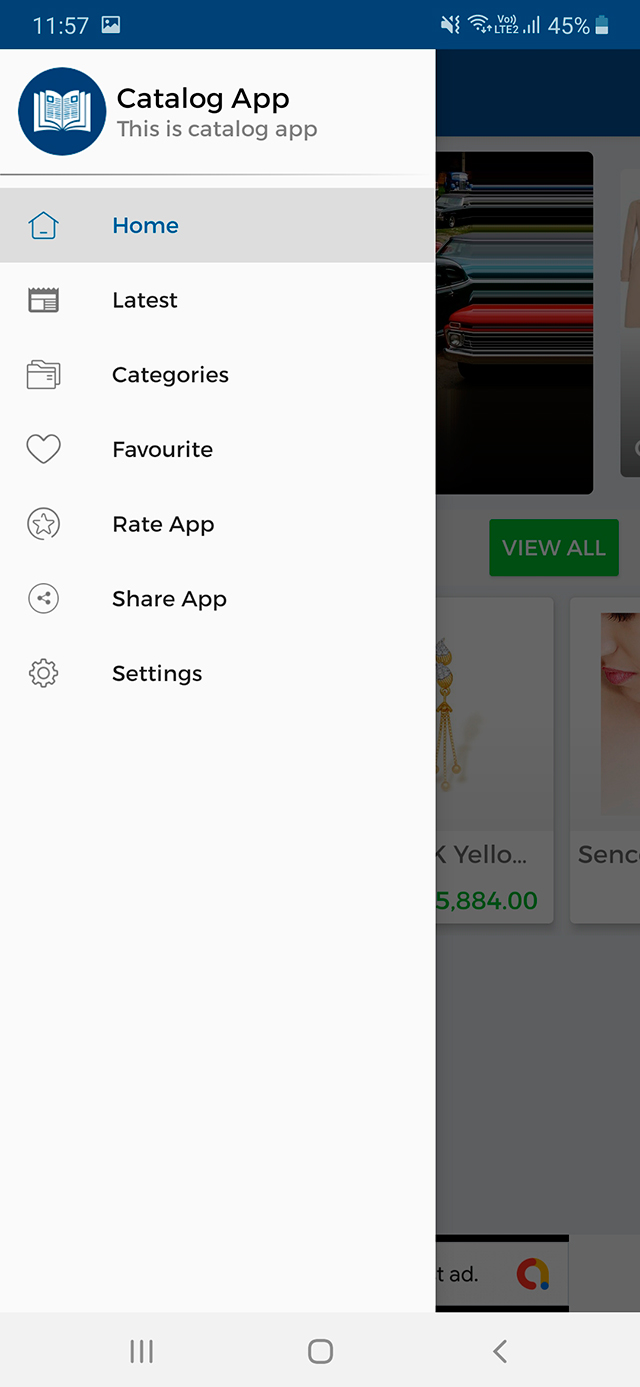A detailed screenshot captured from a catalog app, showcasing its navigation categories and corresponding icons. The top of the image reveals the cellphone's status bar, indicating the time as 11:57. To the right in this navy blue bar, five white icons are visible: Wi-Fi connectivity, signal strength, and battery level displaying 45%. The catalog app itself is prominently displayed, with a navy blue circle featuring an open book icon with visible text on both pages. The app's name, "Catalog App," is written in bold black font, and just beneath it, the text "This is Catalog App" is shown in gray.

Inside the app interface, there are seven navigation categories listed. The first category, "Home," identified by an outlined house icon, is currently selected. The second category is "Latest," represented by a page icon. The third category, "Categories," features an icon of sequential files. The fourth, "Favorite," is denoted by a heart icon. The fifth category is "Rate App," with a star icon indicating a rating feature. The sixth, "Share App," is symbolized by a circular icon with an open angle and dots at each endpoint. Lastly, the settings option is marked by a gear icon.

At the bottom of the screen, a gray bar houses three additional icons: three horizontal bars, a rectangle, and a back arrow, providing further options for navigation and interaction within the app.